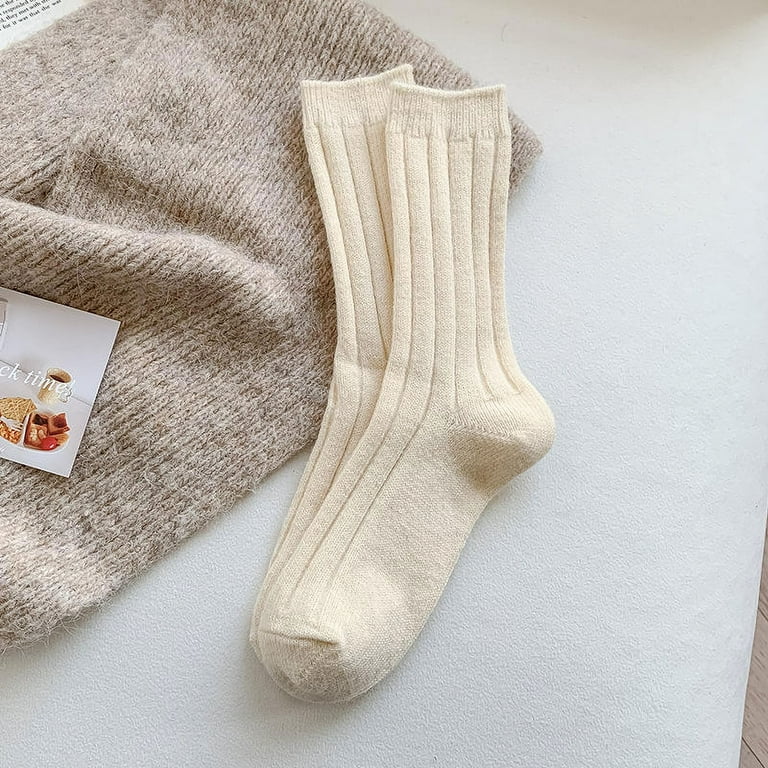This photograph features a pair of cream-colored, ribbed socks with a white elastic band at the top and a gray section at the toe, prominently placed at the center of the image. They rest on a ribbed, slightly fuzzy, grayish-blue knitted scarf that appears almost muted in color. The texture of the scarf suggests it could be a throw or a headscarf, judging by its placement and material. To the left of the socks, partially obscured, is a white card or cord with the term "time" legible on it. The card also contains small photographs of a cup with a dark liquid, a plate of toast with other food items, and a fork, though these details are not immediately noticeable. The overall composition focuses on the socks, which are clean and possibly new, against an understated, neutral-hued background.